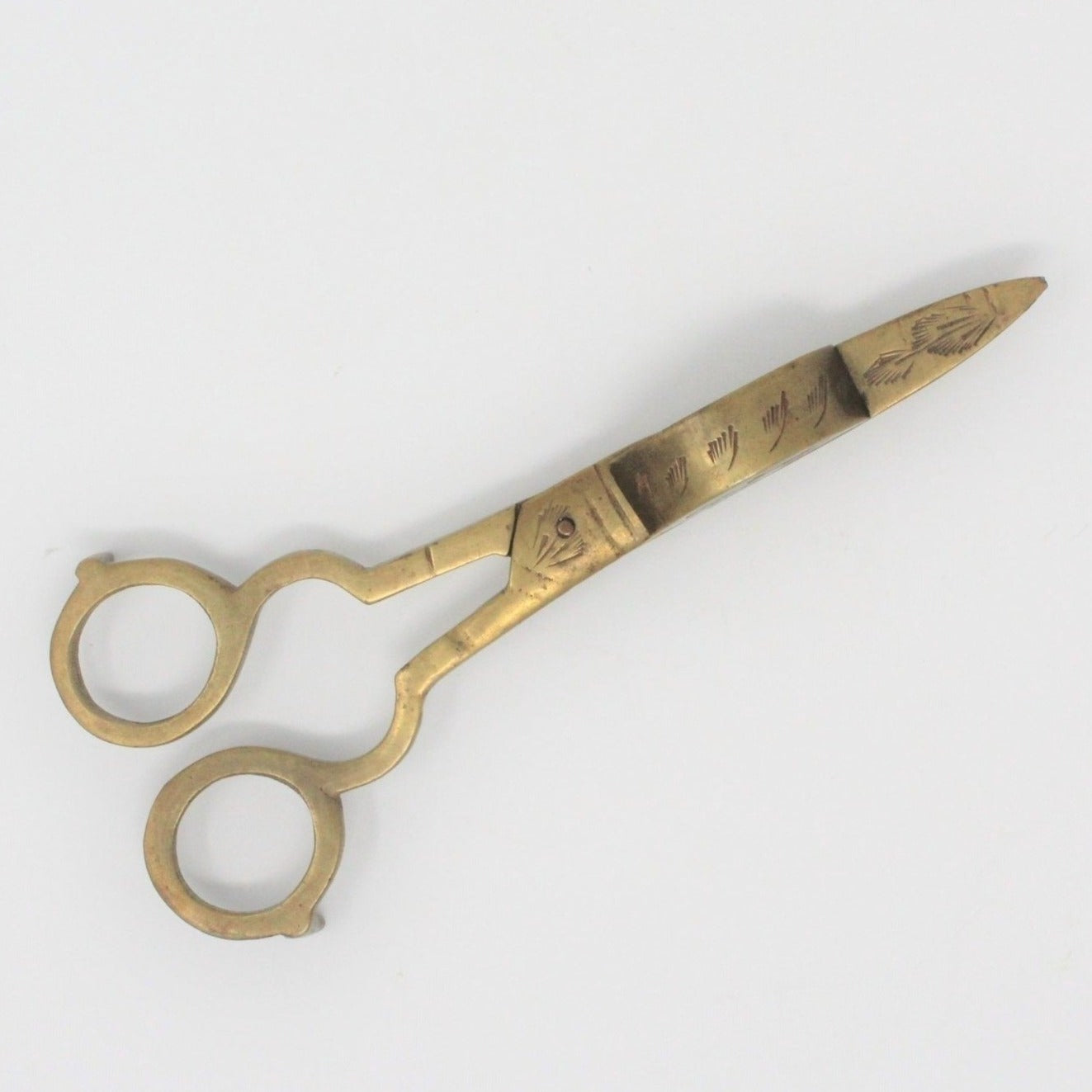This detailed close-up photograph showcases an antique pair of gold or brass scissors diagonally positioned on a flat white surface, with the handles in the bottom left corner and the tips pointing to the upper right. The scissors, likely 100-150 years old, feature intricately engraved designs, including a prominent feather motif that extends from the bottom of the blades up to the central screw. The handles form two small circles, suggesting they are designed for right-handed use. A slight shadow is cast by the scissors onto the background, highlighting their vintage charm and the detailed etchings filled with black that run the entire length of the blades.